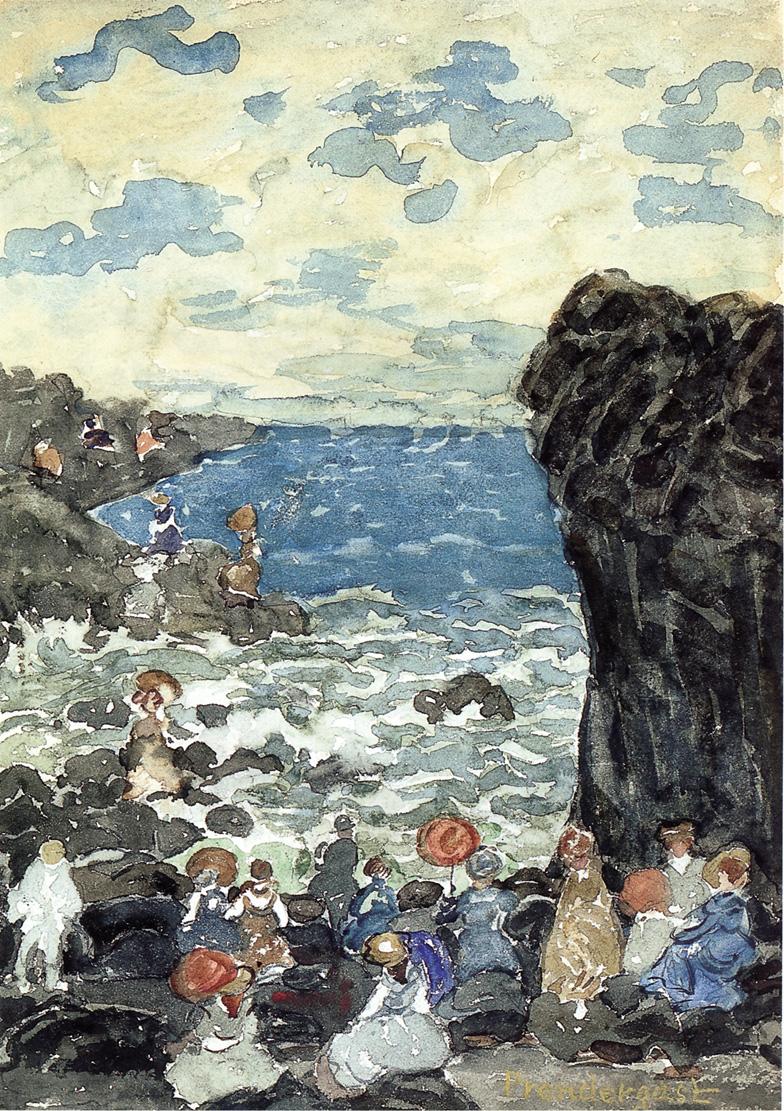The image appears to be a detailed hand-painted scene of a rocky shoreline, likely from an earlier time period based on the attire of the people present. The bottom of the image features several people, predominantly ladies, clad in old-timey outfits such as full long dresses and large hats in various shades of red and brown. They are situated on hilly rocks near the shore, either standing or sitting as they gaze at the crashing waves of the ocean. To the right, there is a towering black cliff, approximately 25 feet high, devoid of any people due to its height. On the left side, there's a smaller cliff where additional people can be seen walking. The sea itself displays a gradient of blue hues, transitioning to whiter and grayer tones near the shore as the waves break. Above the water, the sky is portrayed with a mix of clouds and patches of blue. The colors in the painting comprise a palette of black, various shades of gray, tan, orange, brown, and blues, bringing a sense of depth and atmosphere to the scene. While there is no readable text within the image, a barely discernible signature suggests an artistic touch.